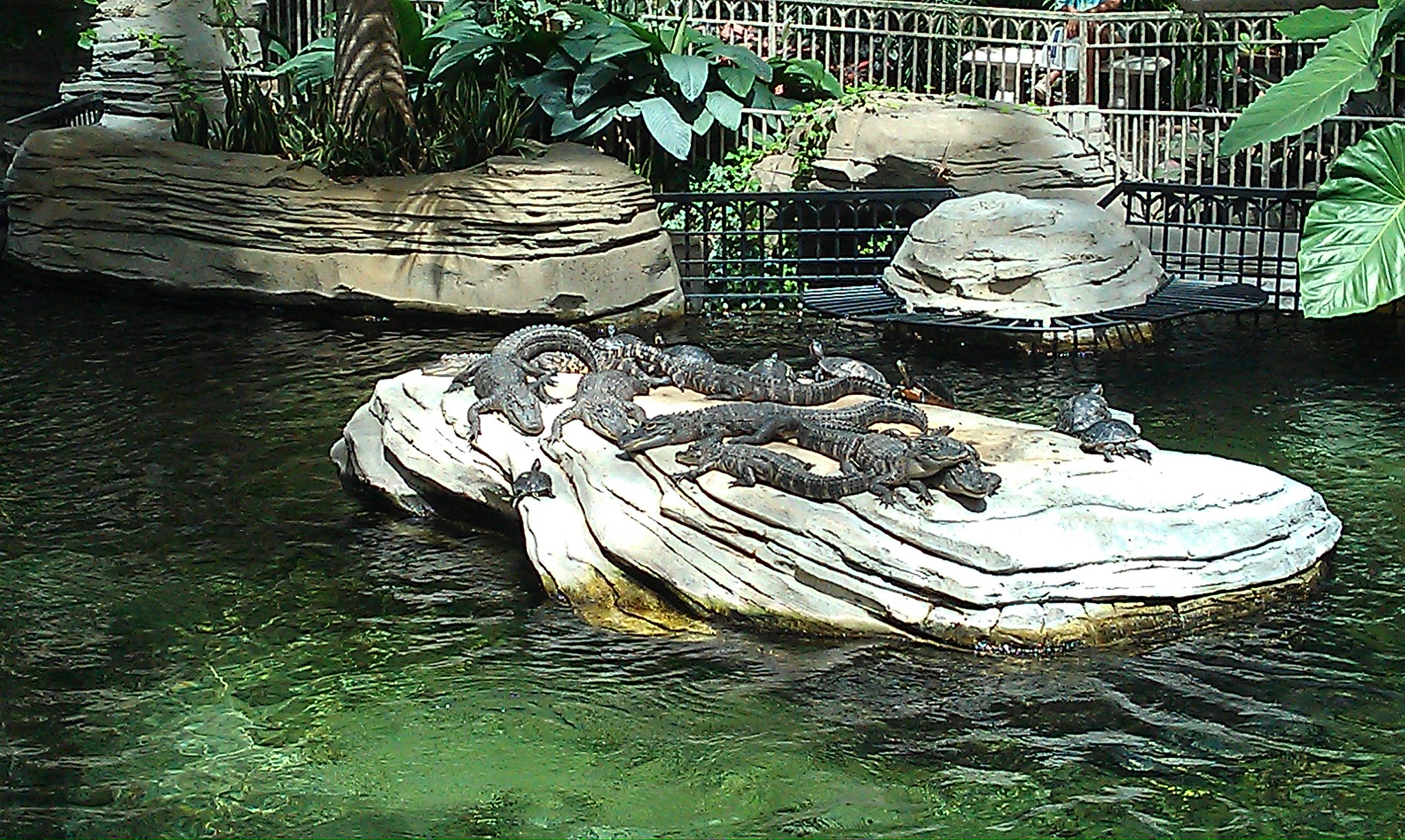This detailed photo appears to be taken outdoors at a zoo, park, or alligator farm, featuring a tropical enclosure with several alligators and turtles. Central to the image is a large cement island, bathed in sunlight, where at least 8 to 10 small alligators lounge and sun themselves. Alongside them, around 8 turtles of various sizes are seen relaxing, with one turtle climbing out of the water. The water surrounding the island has ripples and a greenish tinge in parts. In the background, there's lush greenery with large palm and elephant ear plants, and rocks embedded along the wall. The enclosure is secured by a tall, metal grate fence, both in the foreground and background, ensuring the animals remain safely contained.